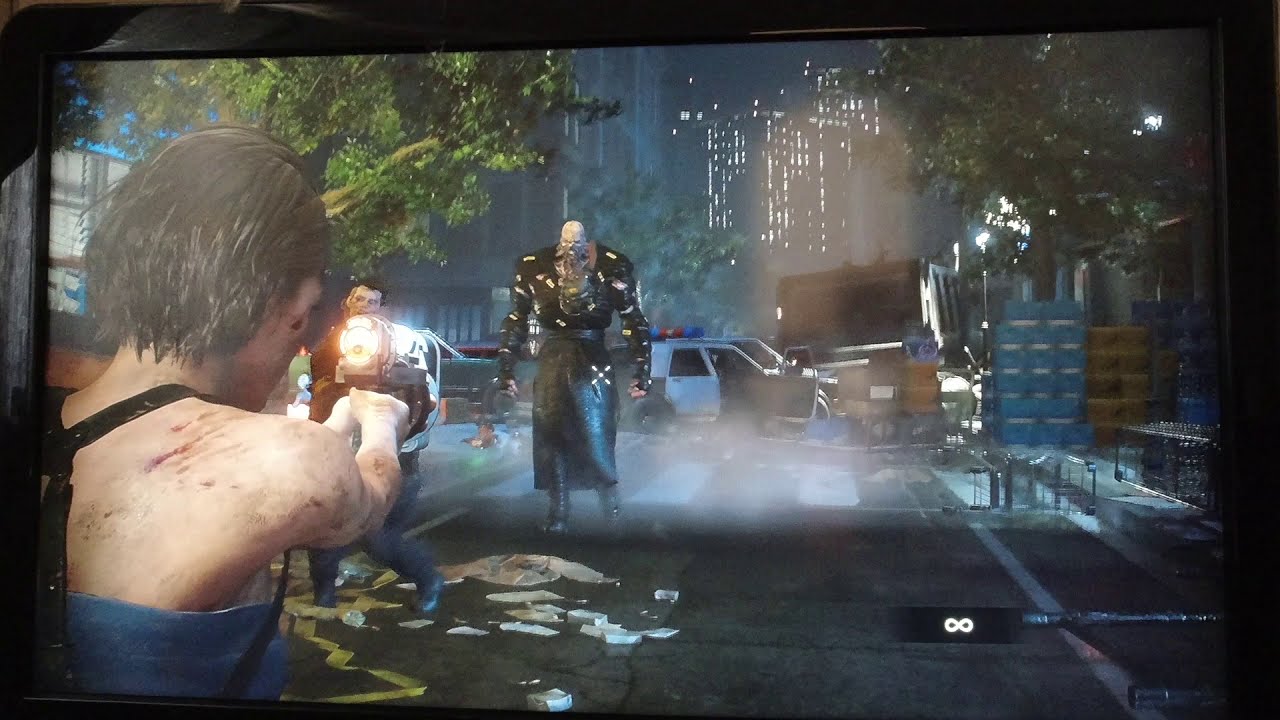In this image, we see a snapshot of a video game being played on a monitor, which dominates 95% of the frame. The focus is on a character in the foreground, viewed from behind, holding a gun. This character has short brown hair and a scratched shoulder, and appears to be aiming at two individuals. 

The central figure in the confrontation is a tall, intimidating man wearing a long black leather jacket with gold flecks, black leather boots, gloves, and a long-sleeved black shirt. He has a bald head, a beard, and his pale complexion gives him a zombie-like appearance. To his left stands what looks like a more typical zombie, with white skin, black hair, short jeans, and boots. 

In the background, there is a police car with its door hanging open, surrounded by various cars and pallets. A large building looms in the distant cityscape. Additionally, an infinity white icon is visible at the bottom right corner of the monitor, adding a subtle touch of game interface to the scene. The overall atmosphere evokes a sense of imminent danger in a post-apocalyptic urban setting.